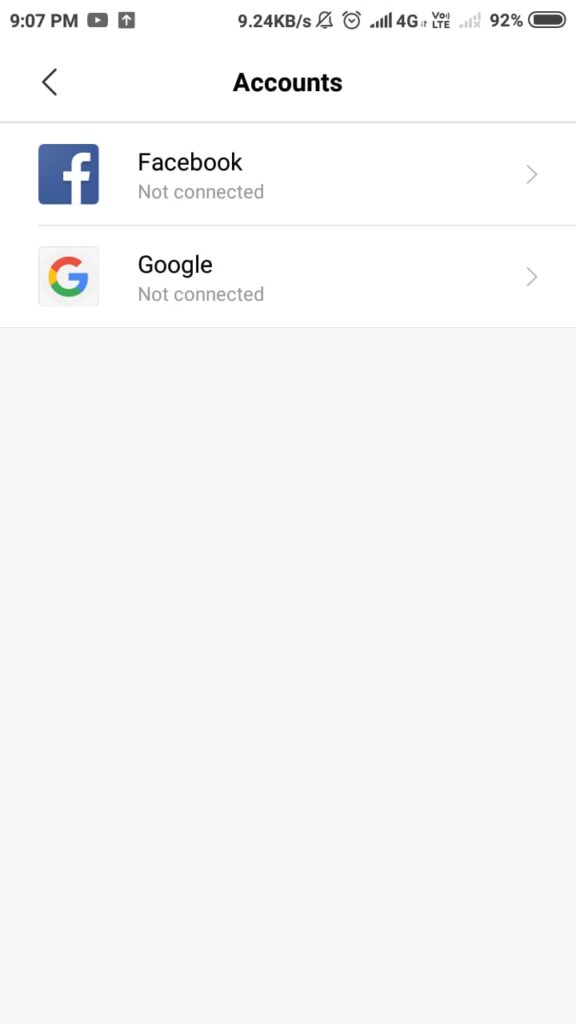Screenshot of a smartphone's account settings page in detail:

The screenshot showcases the account settings page of a smartphone. At the top of the screen, the status bar is visible, indicating it is 9:07 PM. Various icons populate the bar: a YouTube app is open, and an active download is in progress. The phone is connected to a network at a speed of 9.824 KB/s with full 4G service. An alarm is set, the ringer is turned off, and the device's battery is at 92% capacity.

Beneath the status bar, an account header with a back arrow on the left-hand side is displayed. Under this header, there are account connection options: the Facebook logo accompanied by the text "Facebook not connected," and the Google G logo with the text "Google not connected." Both entries have right-facing arrows, suggesting additional menus can be accessed.

The rest of the screen below these options is primarily empty white space, contributing to the simplicity of the image. The screenshot provides a clear glimpse of the phone's settings interface along with a few system notifications.